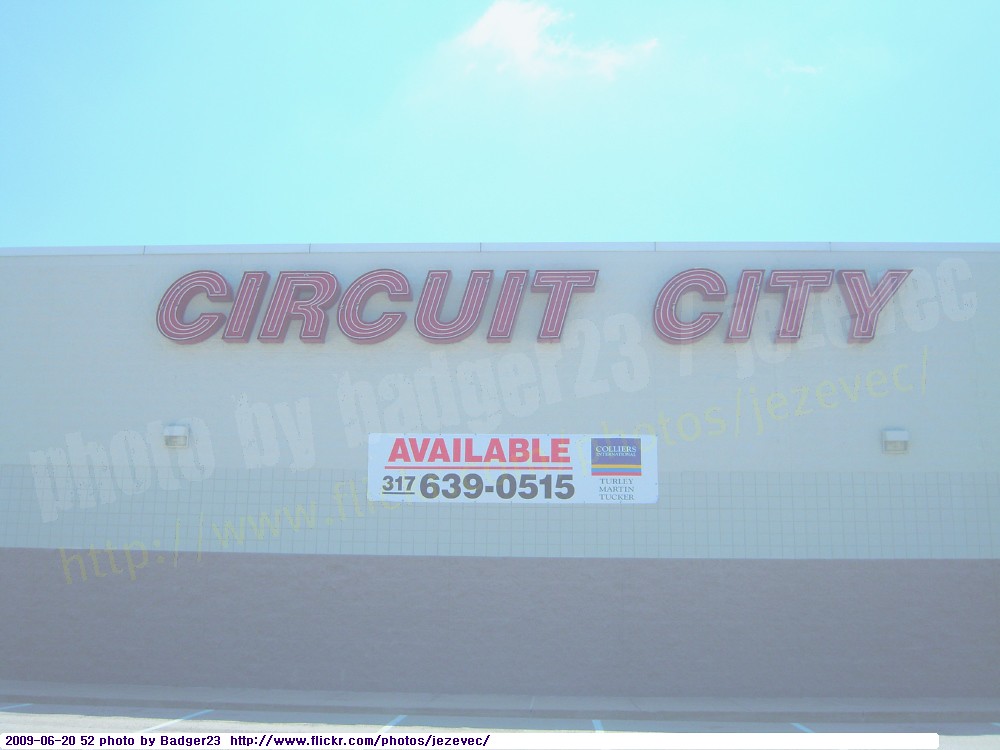This exterior daytime image captures a Circuit City building under a bright blue sky accented by a solitary, fluffy cloud in the center. The building's facade features a light tan color on the top two-thirds, while the bottom third boasts a darker tan brickwork. A gray sidewalk runs along the base of the building, leading to a gray concrete parking lot marked with white lines for parking stalls. Prominently displayed is the Circuit City sign, illuminated by fluorescent lighting, and colored in red. Below the sign is a large white rectangular plaque with red text reading "Available." The plaque also includes a contact phone number, 317-639-0515, and the Realtor's information in black text.